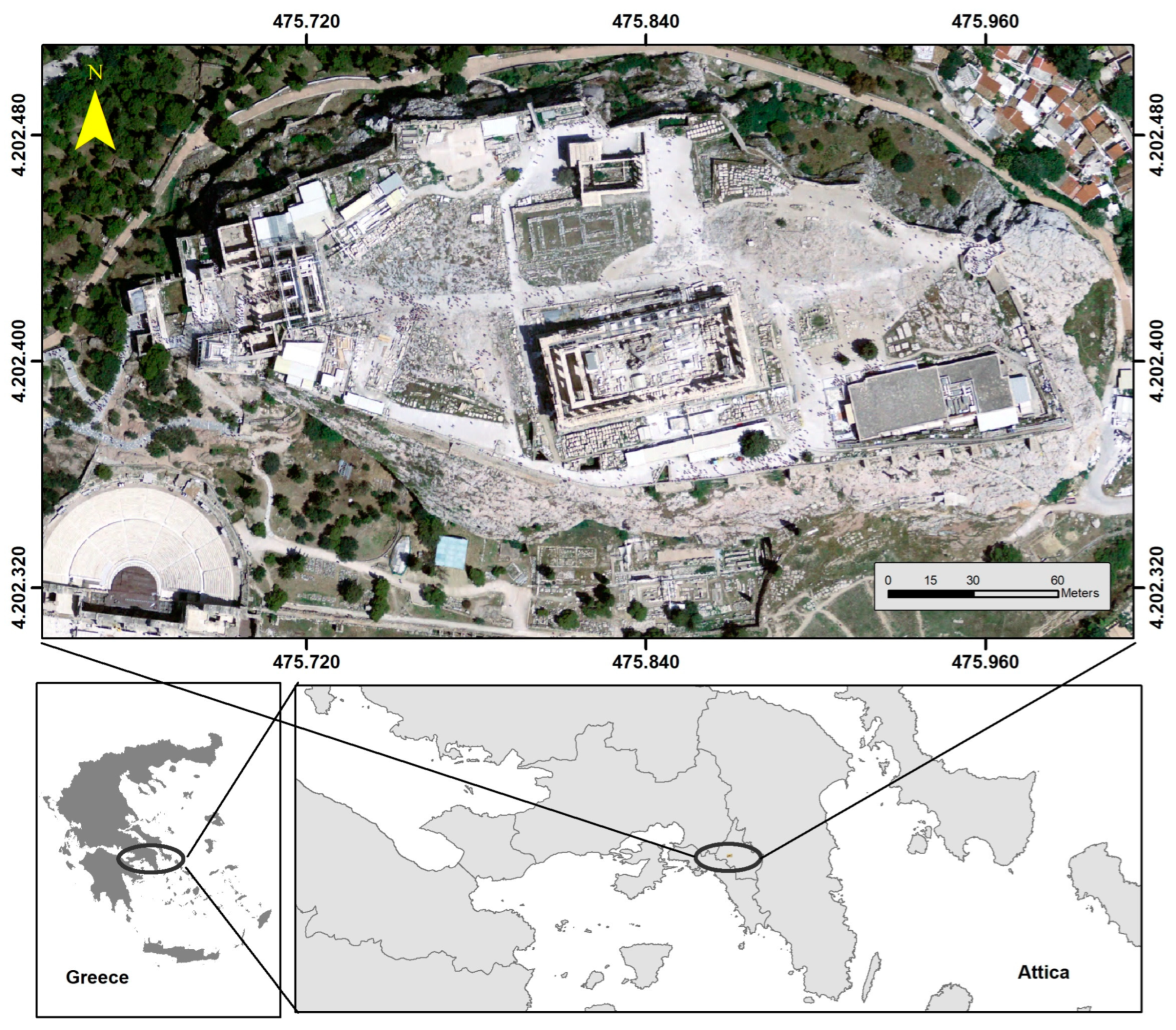The image is composed of three distinct sections, organized into a top and bottom half. The top section is an aerial satellite photograph of the Acropolis Hill, offering a clear, detailed top-down view. The central area of this photograph features several buildings surrounded by a predominantly green landscape with scattered vegetation and trees. Coordinated measurements frame this aerial view, and a distance scale in meters is present at the lower right corner.

The lower half of the image consists of two maps rendered using black lines and varying shades of gray against a white backdrop. The map on the left depicts Greece in a darker gray color within a white background. The map on the right is a closer, detailed view of a region marked as Attica, displaying land in lighter gray with various spires and symbols indicating geographic dimensions. Both maps have areas circled for emphasis. The left map highlights Greece, while the right map, labeled "Attica," focuses on a specific part of the country. 

This composite illustration provides a comprehensive, layered representation of the Acropolis and its contextual geography, valuable for a virtual or self-guided tour of the Acropolis Hill.